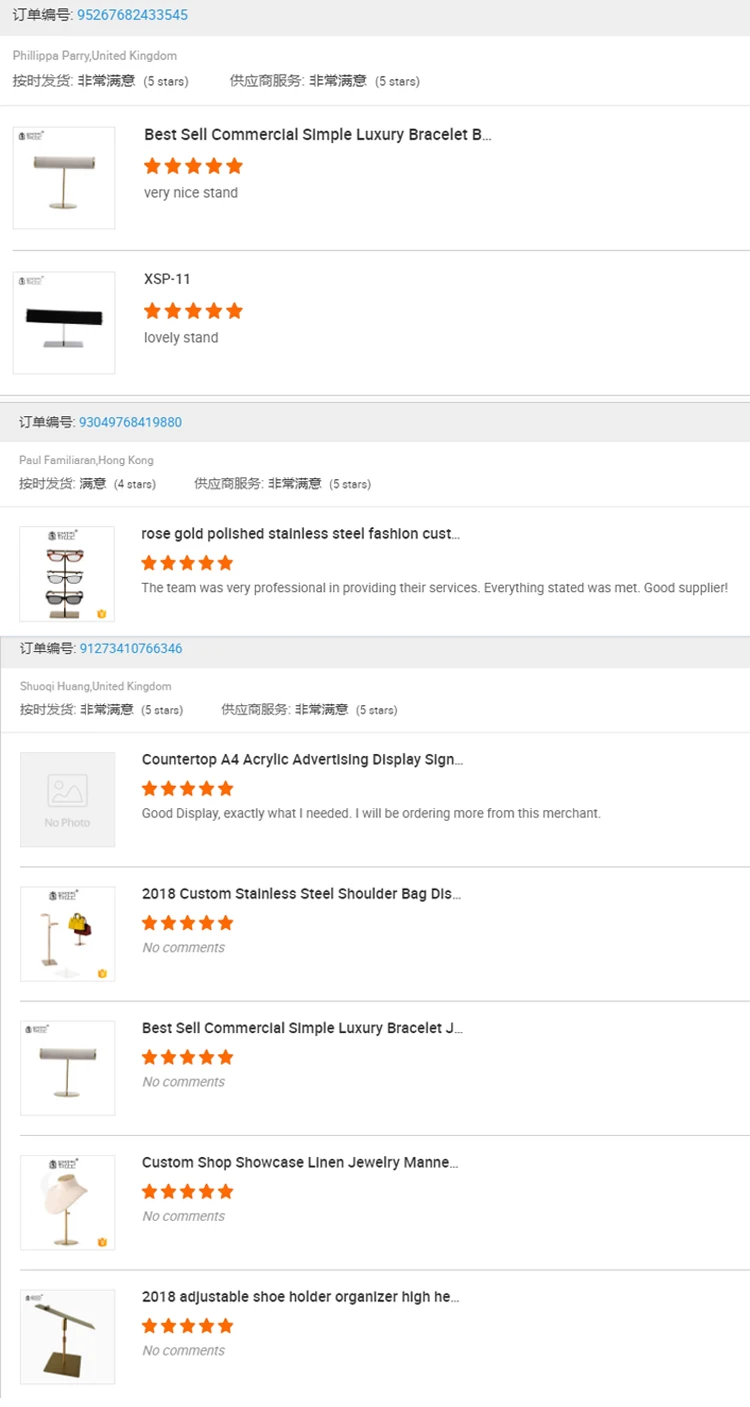The image features a grey banner spanning the top, with Asian characters located in the top left corner, followed by the blue number 95267682433545. Below this, there is small text that reads "Philippe Perry, United Kingdom," accompanied by additional Asian writing and star ratings. 

Below this section, a series of small rectangular images showcase various items:

- An image labeled "Best Sell Commercial Simple Luxury Bracelet".
- An item identified as "XSP-11" which has been rated five stars as a "lovely stand."

Further down the image, another grey banner appears, again featuring Asian writing, followed by another number and a small image labeled "Rose Gold Polished Stainless Steel Fashion."

Yet another grey banner follows, featuring more Asian writing and a number, beneath which there is a listing that begins with a text-only entry for a "Countertop A4 Acrylic Advertising Display Sign." 

The subsequent four items are visualized with images, showcasing:

1. A 2018 Custom Stainless Steel Shoulder Bag.
2. Another "Best Sell Commercial Simple Luxury Bracelet."
3. A Custom Shop Showcase Linen Jewelry.
4. A 2018 Adjustable Shoe Holder Organizer.